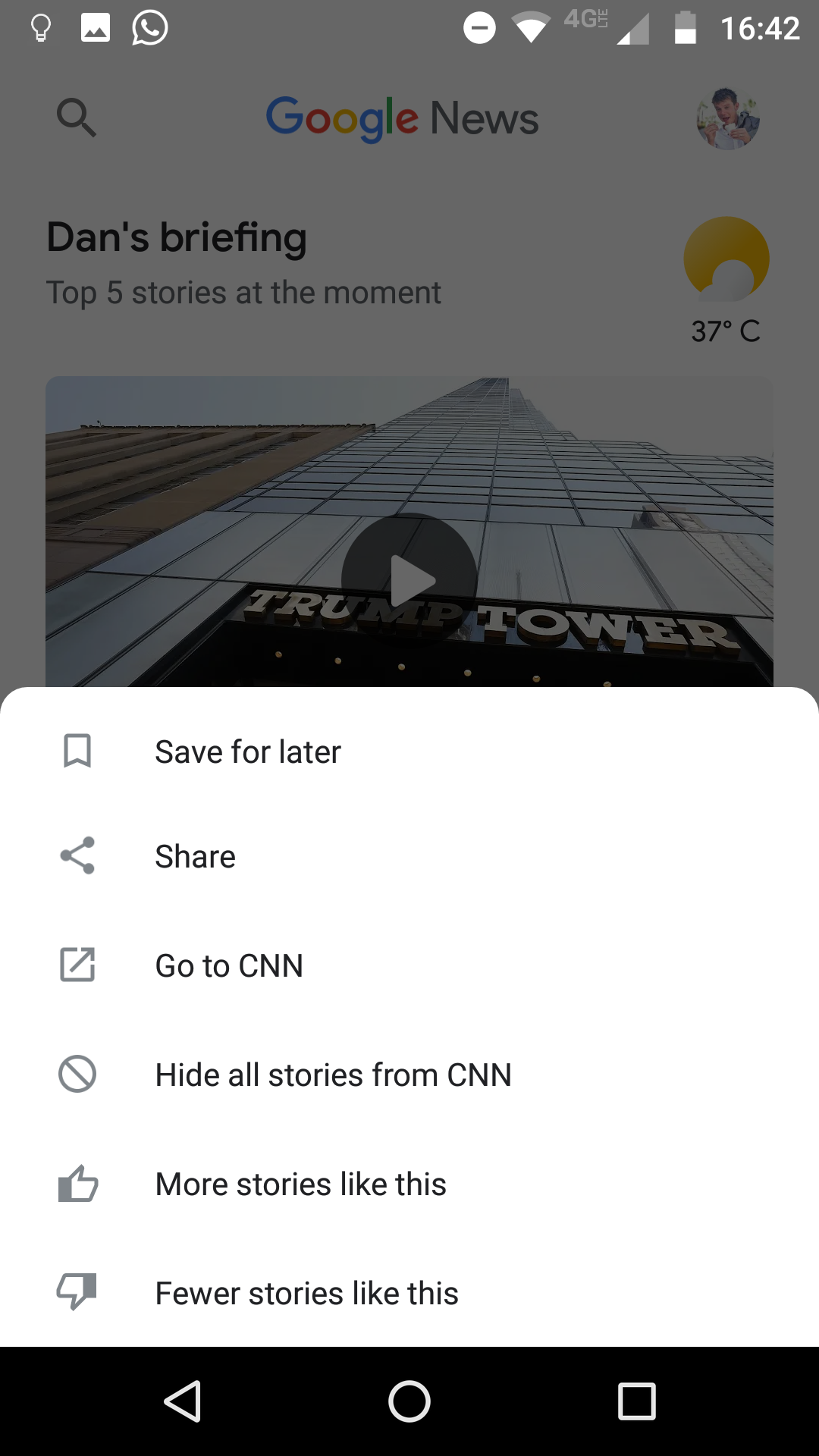The image is a screenshot from a mobile device, displayed in a vertical orientation. At the very top left corner, there are icons for a light bulb, an image, and WhatsApp. On the right-hand side, the status bar indicates the time as 16:42, the battery at approximately 40% charge, and a 4G LTE connection.

The upper half of the screenshot features a gray filter. Underneath the gray filter, there is an interface of Google News, displaying "Dan's Briefing" in black text with a subtitle stating "Top five stories at the moment." Adjacent to this text, on the right, there's an icon of a yellow sun partially obscured by a white cloud, indicating a weather report of 37 degrees Celsius.

The primary story visible at the top is an image of Trump Tower. The building's gray facade and the "Trump Tower" inscription are prominently featured, with the background transitioning into a blue and white sky. A video play button overlaid on the image signifies that this is the static frame of a video related to the top story in the news feed.

Below the main story, there is a pop-up white box presenting a series of interaction options for the user. These options include: "Save for later," "Share," "Go to CNN," "Hide all stories from CNN," "More stories like this," and "Fewer stories like this."